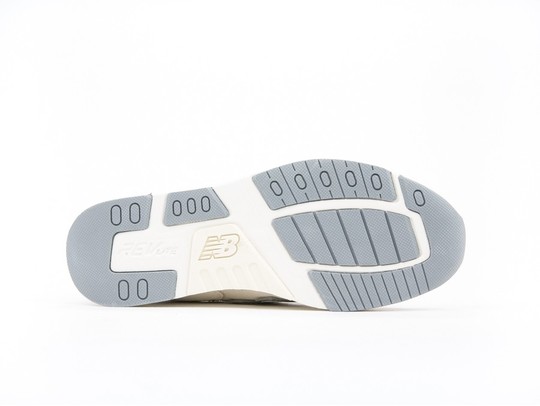The image depicts the sole of a left New Balance shoe, showcased on an eggshell white background. The shoe is positioned slightly off-center, though primarily occupying the middle of the frame. The sole features a combination of white and gray colors, with reinforced areas around the toe, heel, and insole. Prominently displayed on the sole is the New Balance logo (NB) in a beige or gold hue. The textured bottom includes a pattern of circular elements, specifically 11 around the outer edge and 2 near the inner heel. The brand new shoe has a clean appearance with a small sliver of its white or ivory upper body visible. The absence of additional text or elements suggests it is a professional photograph likely intended for a shoe collector, store, or online retail site, emphasizing the realistic and detailed representation of the product.